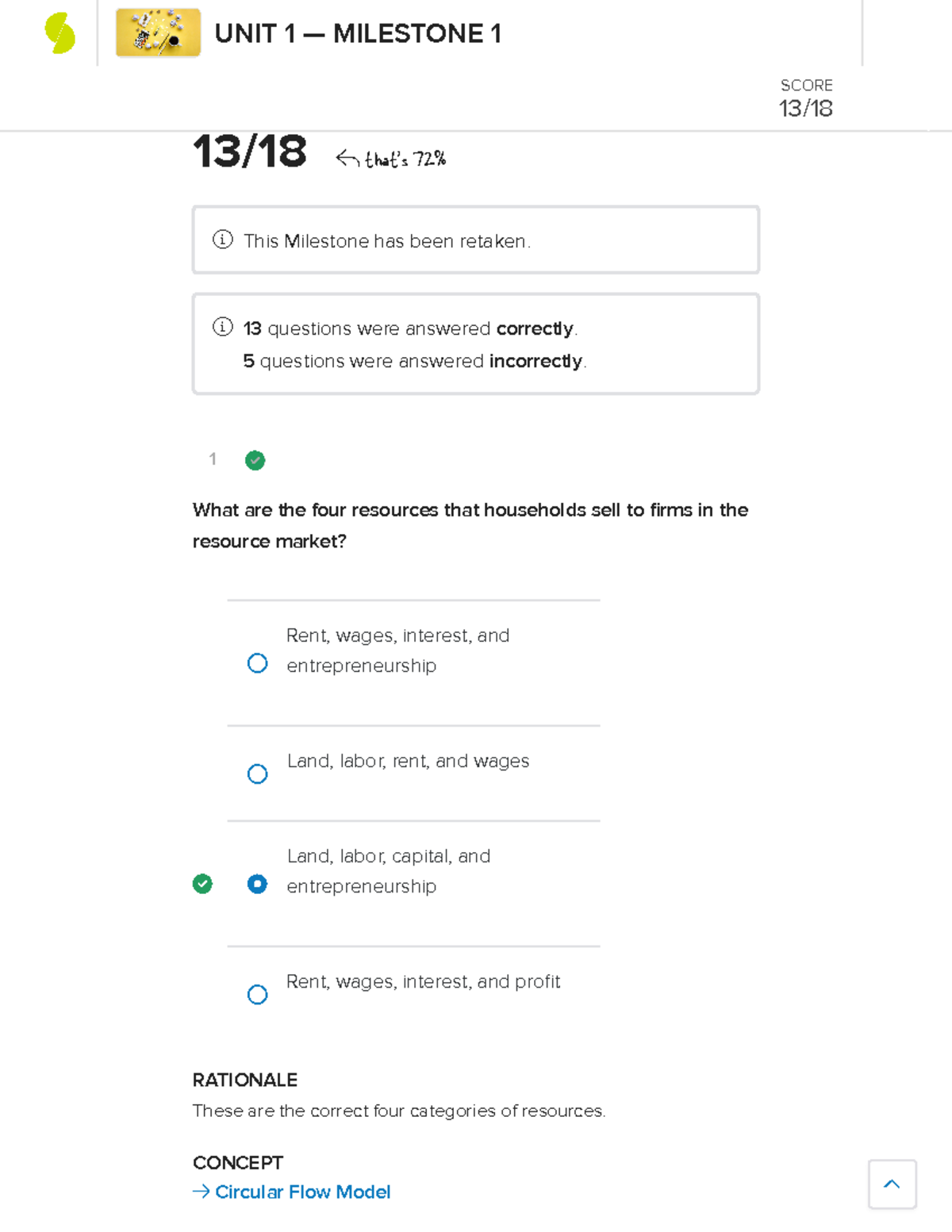The image, titled "Unit 1 - Milestone 1," appears to be a progress overview for an educational milestone. In the top-left corner, a rectangular box with a yellow background displays an assortment of calculators and other electronics. Just below this image, the text "13/18" is visible, followed by a rightward arrow indicating a score of 72%.

Two distinct text boxes are featured below this score. The top box reads, "This milestone has been retaken," accompanied by a circular icon with an 'I' on its left side. The second box states, "13 questions were answered correctly. 5 questions were answered incorrectly," with another 'I' icon to its left.

Centrally located in the image, a number "1" with a green checkmark signifies a correctly answered question. The question posed is, "What are the four resources that households sell to firms in the resource market?" displayed beneath it. Four answer options, each within blue-outlined bubbles, are listed as follows:
1. Rent, wages, interest, and entrepreneurship.
2. Land, labor, rent, and wages.
3. Land, labor, capital, and entrepreneurship.
4. Rent, wages, interest, and profit.